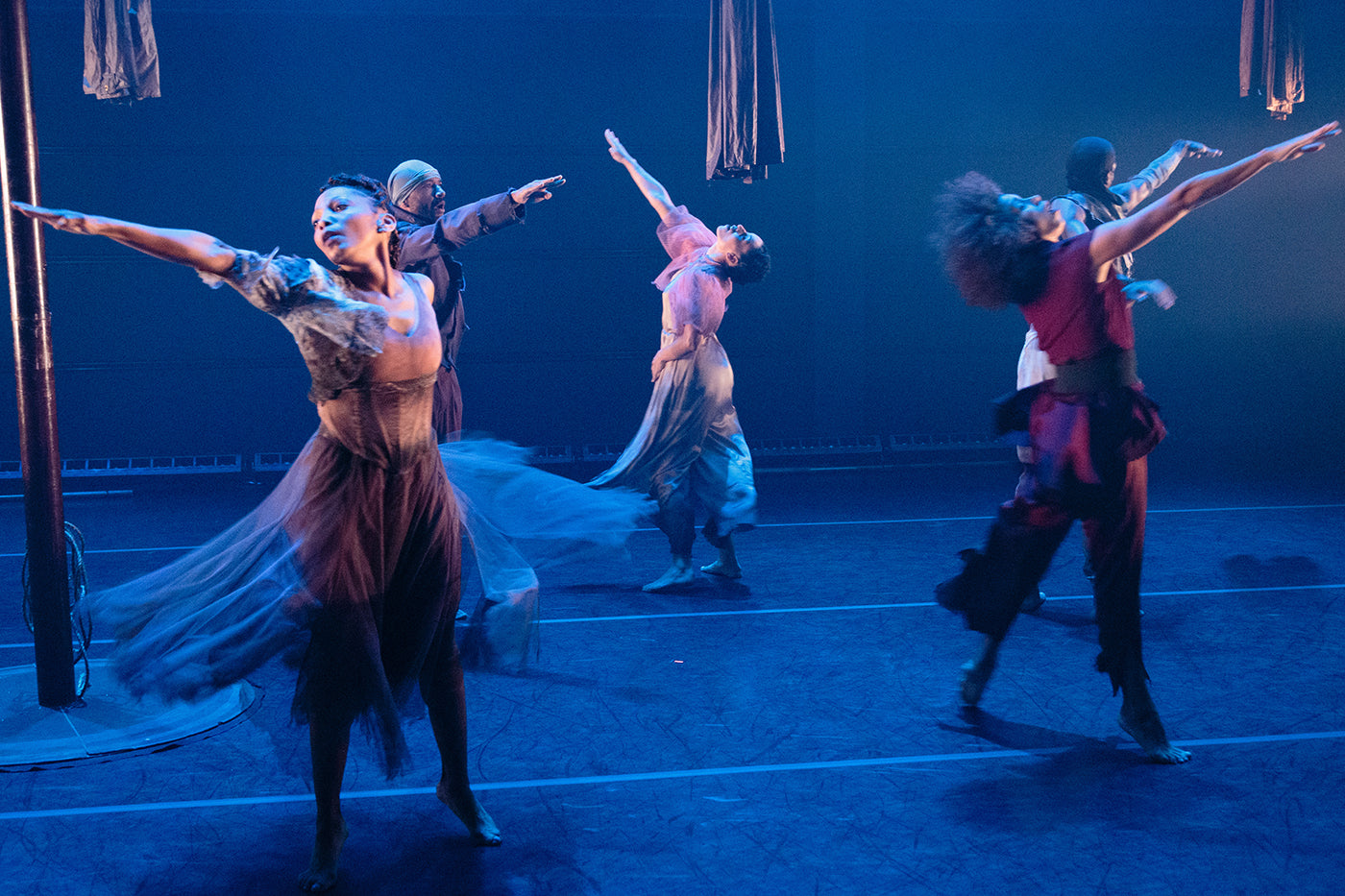This image captures a poignant dance performance inspired by Les Miserables. The stage is set against a dark black background and a dark black floor, accentuated by white stripes running across it. Suspended from the unseen ceiling are three white drapes, framing the scene dramatically. The stage design also includes three visible curtains.

In the center of the composition are five dancers, three women and two men. The women wear either burgundy or pink tops and bottoms with see-through skirts, and the men, though partially obscured, are dressed in similarly tattered, period-appropriate attire, complete with skull caps. All dancers appear to be African American, contributing to the emotive depth of the performance.

Every performer strikes a similar pose, with one arm extended upward towards the ceiling, their eyes following their gesture, creating a sense of yearning or distress. Despite their expressive postures, the dancers' faces remain neutral, evoking a solemn mood.

The stage is well-lit, casting a bright light that enhances the dramatic contrasts of the scene, yet maintaining a dark and somber atmosphere. Off to the left, almost out of sight, a pole adds a subtle, intriguing element to the composition. This meticulously detailed image combines elements of modern dance with evocative historical references, capturing a moment of powerful expression and collective movement.